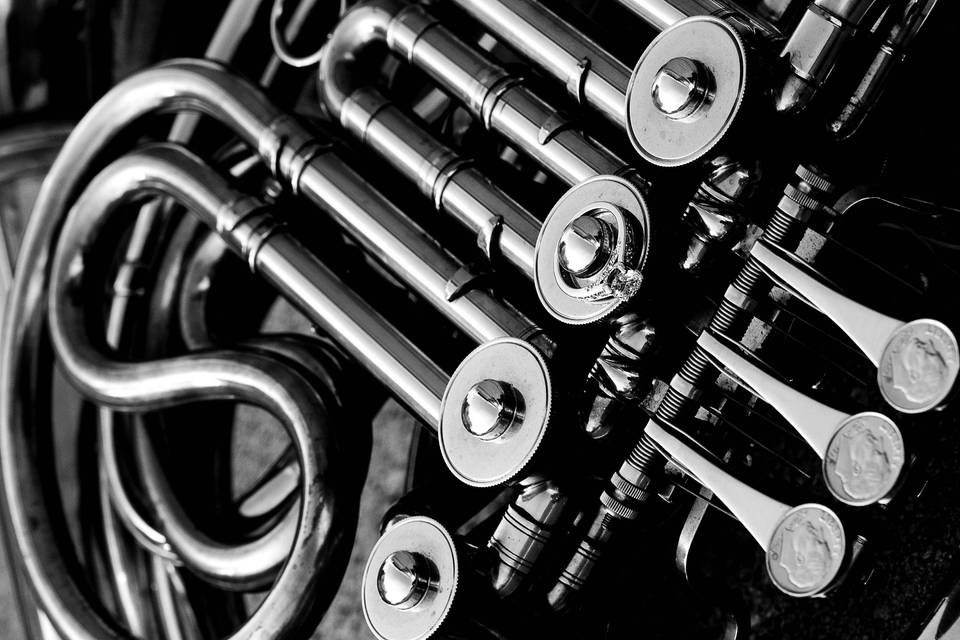This black and white photograph showcases a sleek, metallic mechanical device or musical instrument, characterized by a series of smooth, intertwining silver or platinum tubes and valves. The intricate design lacks visible gears, instead presenting a seamless and polished appearance, with the tubes curling into an obscure black background. Dominating the bottom right corner are three finger pedals, each adorned with a dime. Central to the composition is a diamond ring, suspended on one of the round disc rivets, adding a perplexing element that suggests a potential proposal setup but lacks further context. The high contrast between the silvery components and the dark background emphasizes the intricate details, making the image both striking and enigmatic.